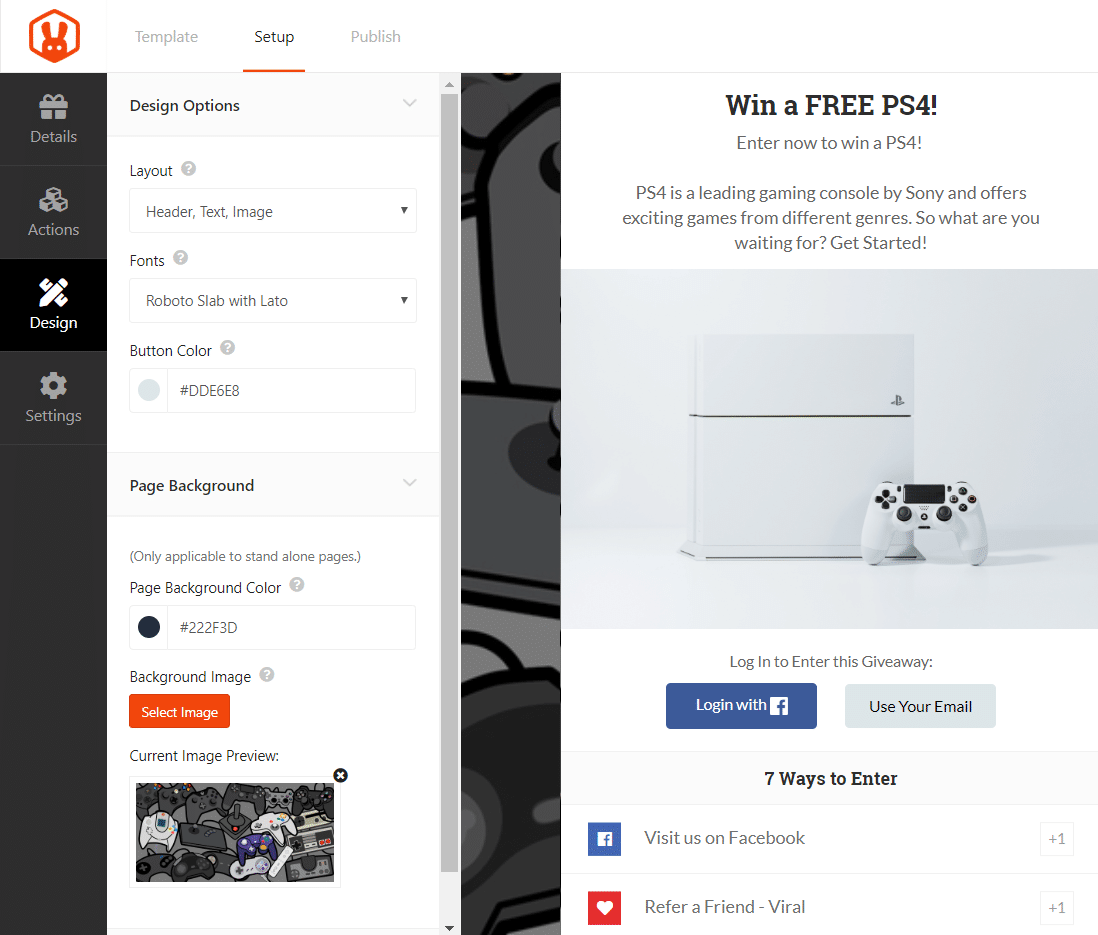Screenshot of a webpage featuring a design and settings interface. The top left corner displays an orange hexagon with a rabbit and white eyes. On the left, a vertical gray bar contains various icons and text: a present icon labeled 'Actions,' three dice, a pencil crossed by a ruler for 'Design,' and a gray gear for 'Settings.'

The vertical column titled 'Design Options' includes sections for Layout, Header, Text, Image, Fonts with 'Roboto Slab' and 'Lato,' Button Color with a code #DDF6F8, and Page Background with a color code #222F3D, noting it's applicable only to standalone pages. An orange 'Select Image' button appears below, along with a preview of a current image showing colorful cartoon video game consoles.

On the right, text promotes a giveaway with "Win a Free PS4. Enter now to win a PS4," emphasizing Sony's PS4 as a top gaming console with diverse exciting games. Beneath the text is an image of a white PS4 console.